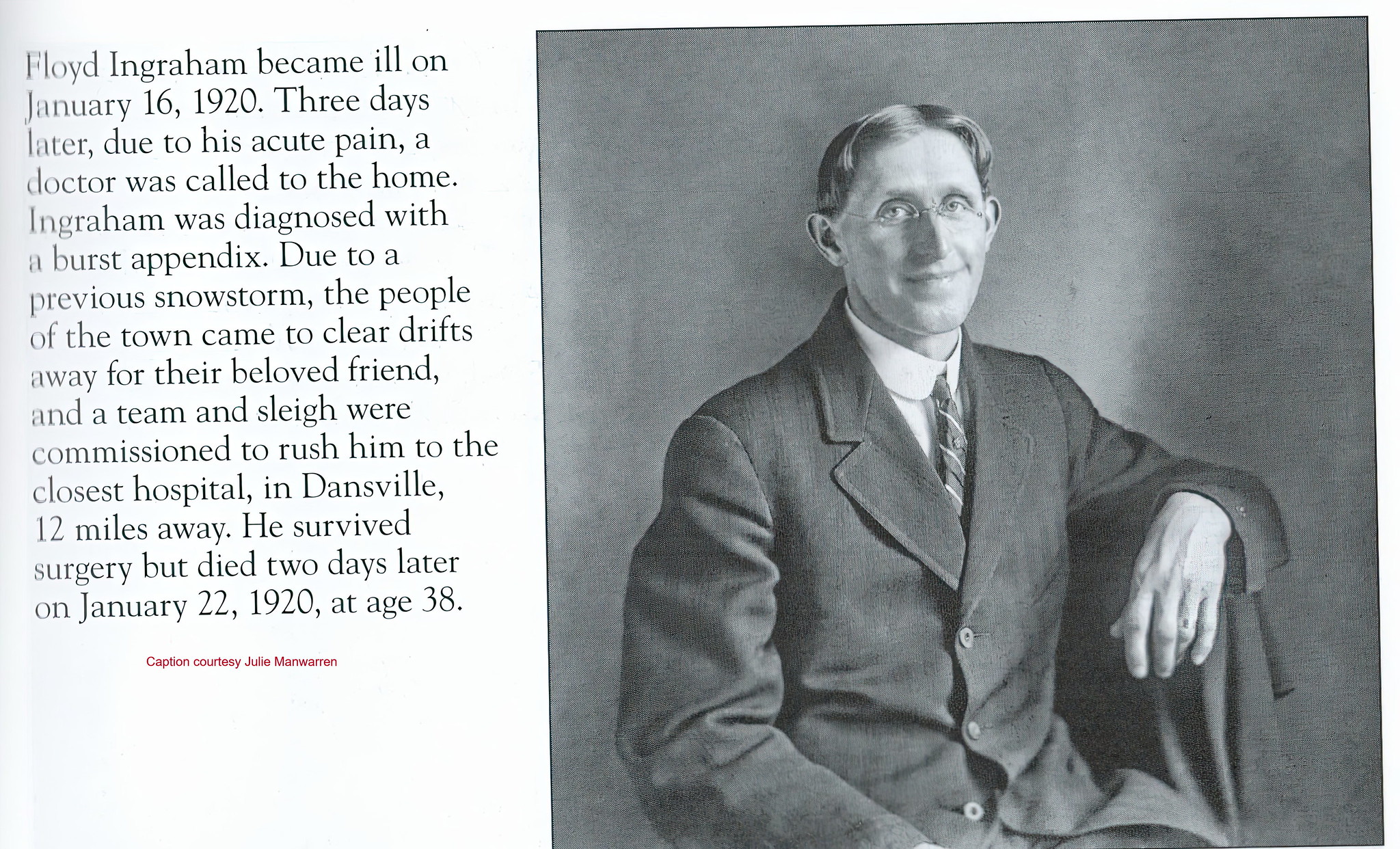The black and white image depicts a middle-aged man with short, dark hair and old-fashioned spectacles, sitting sideways on a chair with his left arm draped over the chair's back. He is smiling slightly and looking towards the camera. The man is wearing a black sport jacket, a multicolored tie, and a white undershirt. His hair is parted in the middle. To the left of this portrait, there is a block of text in black font that reads: "Floyd Ingram became ill on January 16th, 1920. Three days later, due to his acute pain, a doctor was called to the home. Ingram was diagnosed with a burst appendix. Due to a previous snowstorm, the people of the town came to clear drifts away for their beloved friend, and a team and sleigh were commissioned to rush him to the closest hospital in Dansville, 12 miles away. He survived surgery but died two days later on January 22nd, 1920, at age 38." Below this text, another line in red font reads: "Caption courtesy Julie Manwarren."